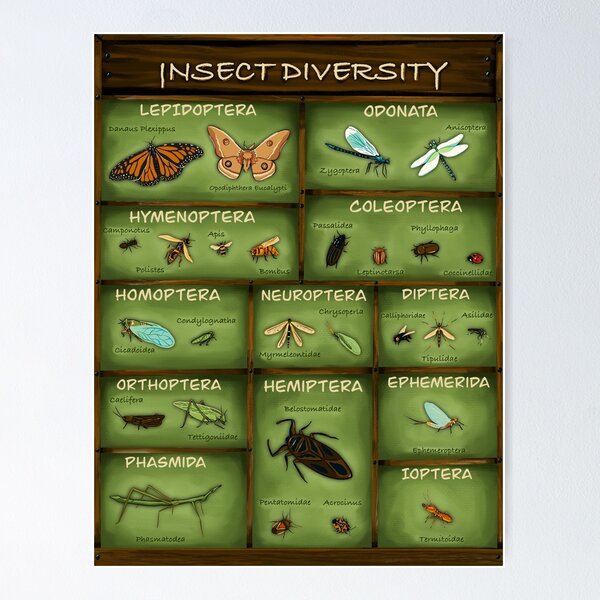The image depicts a highly detailed poster centered around insect diversity, prominently titled "Insect Diversity" in white text across the top. The poster is bordered with a design resembling a wooden frame and is divided into various sections, each with a green backdrop highlighting different types of insects. Detailed sketches of butterflies, dragonflies, beetles, bees, wasps, and an assortment of other insects fill these sections, with many areas featuring multiple species. Each insect is labeled with its Latin name, such as Lepidoptera for butterflies and moths, Odonata for dragonflies, Coleoptera for beetles, and Hymenoptera for bees and wasps. The insects are illustrated in natural colors, simulating their appearance in the wild. This educational poster, likely suitable for a biology classroom, offers a visually appealing guide to identifying and learning about the diverse world of insects.